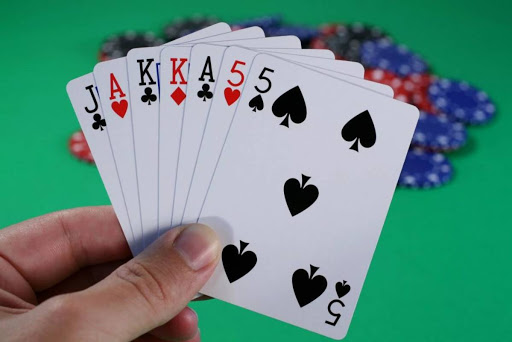In the bottom left corner of the image, a person's left hand is positioned prominently, clasping a set of traditional playing cards. The thumb is featured prominently, with the other fingers curled behind it, holding the cards. The sequence of cards from left to right includes a Jack of Clubs, Ace of Hearts, King of Clubs, King of Diamonds, Ace of Clubs, Five of Hearts, and Five of Spades. These cards are standard white with classic designs: black for the spades and clubs, and red for the hearts and diamonds. The five of spades is the most visible card on the right, showcasing five black spades. The background depicts a green velvet poker table, providing a traditional and elegant setting. Additionally, there is a pile of poker chips in blue, red, and black, each adorned with white indentations along their outer edges.